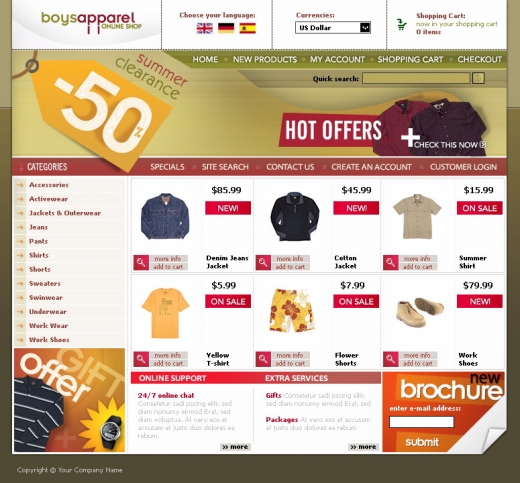Screenshot of a Digital Coupon Interface

At the very top of the image, there are two white sections. The left section displays "Boys Apparel Online Shop," and the right section allows users to choose their language, showing icons of the UK flag, the German flag, and the Spanish flag. Next to this is a currency drop-down menu, where the selected currency is the US Dollar. The shopping cart icon on the far right indicates "0 items."

Below this header is a green navigation bar with menu items: Home, New Products, My Account, Shopping Cart, and Checkout. Beneath the navigation bar is a "Quick Search" feature.

To the right, there is a banner that reads "Hot Offers" in white text over a red bar. Below this, images of a dark red shirt and a dark purple shirt are displayed, with a plus sign and the text "Check This Now."

On the left, there is an orange tag with "-50%" written on it, indicating a discount. Above this tag, "Summer Clearance" is prominently displayed.

The central section of the interface showcases various items on sale, each with an accompanying image. The items listed are:
- Denim Jeans
- Jackets
- Cotton Jacket
- Summer Shirt
- Yellow T-Shirt
- Flower Shorts
- Work Shoes